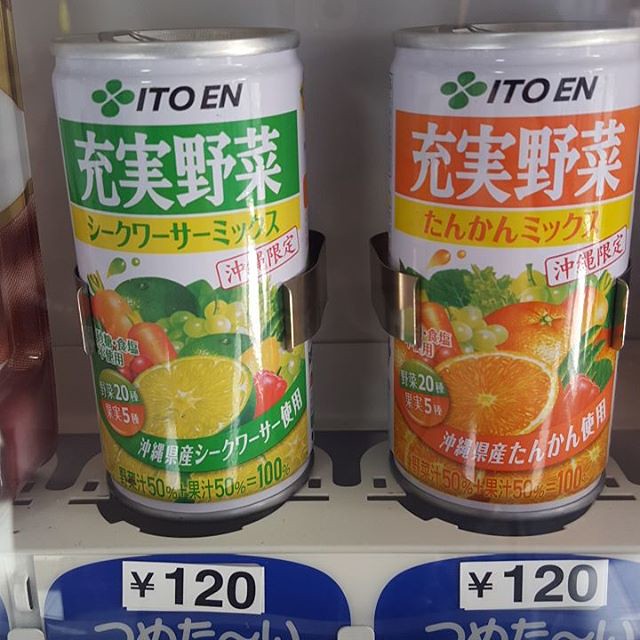This is a detailed close-up photograph of two aluminum beverage cans inside a vending machine in Japan. The cans are held in place by metal claw-like contraptions. At the bottom of the image, there are white labels with black font indicating the price, which is 120 yen. Beneath the price, each label also includes the word "sumetai," meaning cold in Japanese. On the left is a green can featuring a design with lime slices and other fruits, identified as a lime-flavored drink. The on the right is an orange can with a design showcasing orange slices and other fruits, identified as an orange-flavored drink. Both cans are branded with "ITO EN" (I-T-O space E-N) at the top.